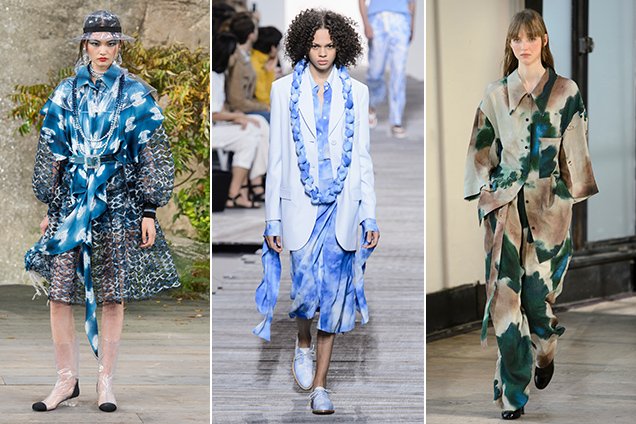This triptych showcases three models in distinct and stylish outfits, each set against different backgrounds. 

The leftmost image features a female model, who appears to be of Asian descent, dressed in a layered blue dress adorned with white graphic elements resembling doves or birds. Her ensemble is completed with a black hat that has a translucent bill, clear knee-high boots with dark black tips, and silver jewelry featuring black and white beads. She is posed outdoors on a gray ground with a green tree bearing yellow leaves visible in the background.

The central image captures a Black model with frizzy dark hair, styled in a long blazer paired with a white and blue dress. She wears light blue shoes and a Hawaiian-style lei made of the same blue and white material. The model is walking on a wooden pathway, likely at a fashion show, with audience members seated in the background. Among them are a woman in white with black sandals, a man in a tan coat with blue jeans, and another person in yellow. A man can be seen walking behind the model, dressed in blue and white attire.

The rightmost image presents a model dressed in a suit featuring beige, brown, and green hues, with green pants and black shoes. This outfit displays a unique pattern that resembles ink spreading on a beige background. This model is walking on a brown ground within an indoor setting, which features white walls with black trim and a window framed in black. 

The combined presentation of these images creates a vivid and dynamic depiction of diverse fashion styles and settings, likely captured during a fashion week or show event.